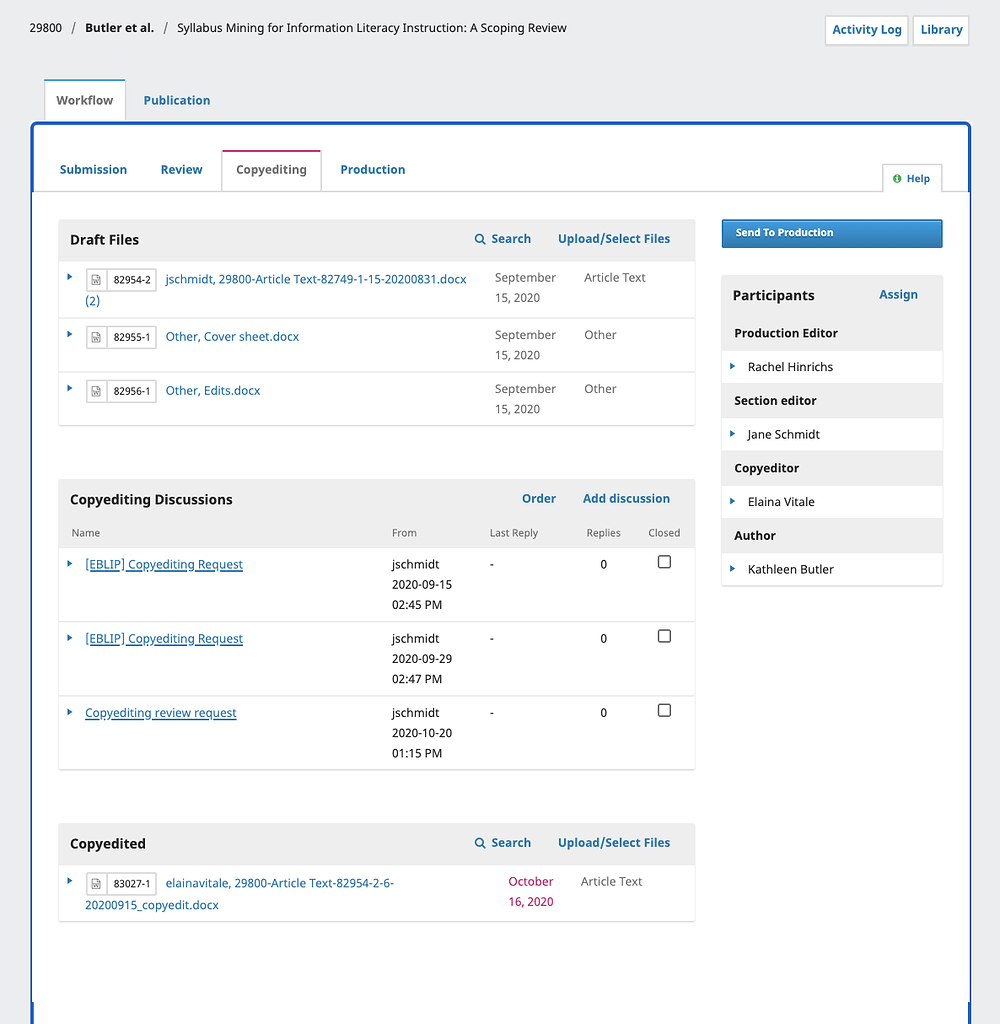The image depicts the detailed interface of an academic tool, presumably a manuscript management system, designed for writing and reviewing scholarly work. Central to the image is text that reads: "29800 / Butler et al. / Syllable Syllabus: Mining for Information Literacy Instruction – A Scoping Review." To the right of this text are two buttons with a gray background and blue text: the first button is labeled "Activity Log," and the second is labeled "Library."

Below this section, on the left side of the interface, there are two highlighted sections: "Workflow" and "Publication." The "Workflow" section is selected, displaying a white background outlined in blue. Within this area, a header provides several options: "Submission," "Review," "Copyediting," and "Production." Currently, "Copyediting" is selected, as indicated by a red border on its top edge. To the right of this header, there is a help button featuring a green circle with a white "i" (information icon).

The layout of the "Copyediting" section is divided into two main columns. The left column, which occupies approximately 60-70% of the space, includes several sections:
1. **Draft Files**: A gray header with black text and three list elements in blue.
2. **Copyediting Discussions**: A similar gray header with three list elements.
3. **Copyedited**: A section featuring one list element at the bottom.

The right column, significantly narrower, is titled "Participants". It contains sub-list elements indicating roles, such as "Production Editor," followed by the name of the individual with a blue drop-down arrow.

Each section and list element appears to provide structured data management and collaborative options, indicative of a comprehensive tool for scholarly publication workflows.